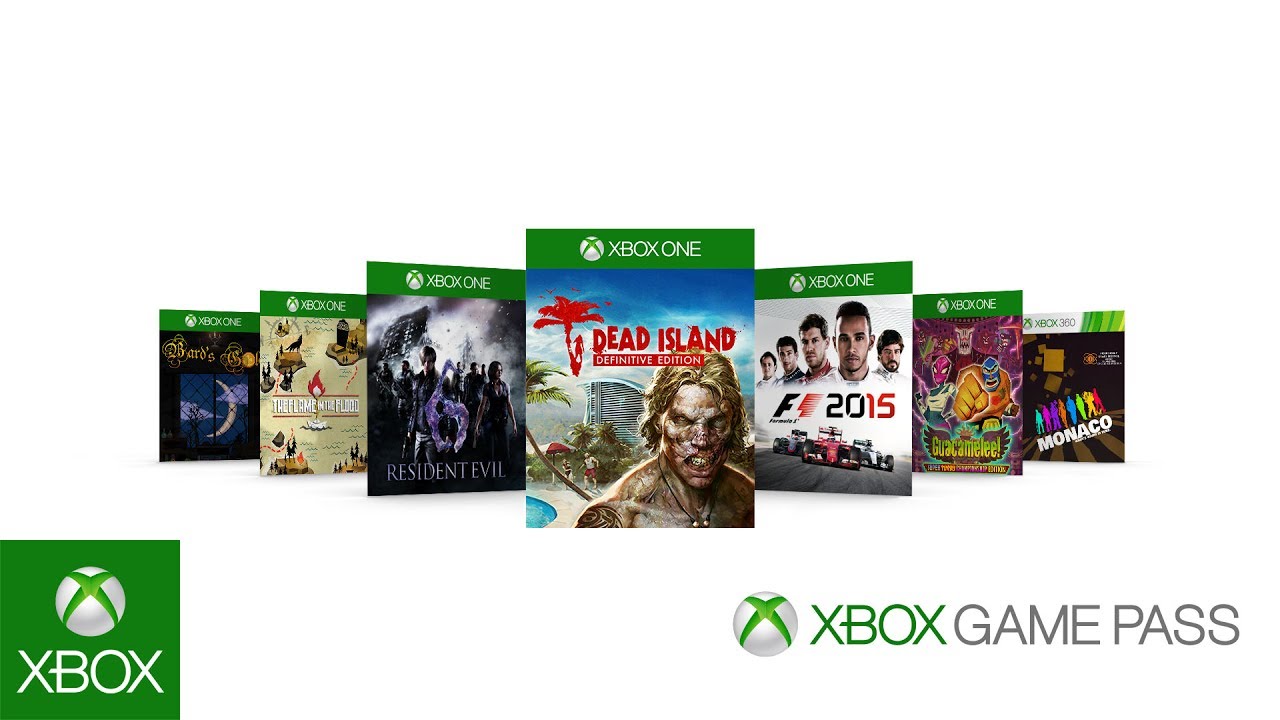The image is an advertisement showcasing a selection of Xbox games. In the bottom left corner, there's a green square featuring the white Xbox logo and the word "Xbox" in white font. Adjacent to this, there's another logo with the iconic Xbox ball, with "Xbox" in green font followed by "Game Pass" in gray, uppercase letters.

The advertisement displays seven game covers:

1. The first game's title is partially visible, with "Xbox One" clearly marked, but the specific game title is unreadable.
2. The second game is also an Xbox One title, featuring artwork that depicts castles and fire, suggesting a fantasy or medieval theme.
3. The third game is "Resident Evil," recognizable as another Xbox One game.
4. Positioned in the center is "Dead Island Definitive Edition" for Xbox One, showcasing a zombie at a beach resort scene.
5. To the right of the center, the game "F1 2015" is listed, clearly indicating a Formula 1 racing theme.
6. The next two games are partially obscured but are part of the Xbox One collection.

Overall, the advertisement emphasizes the diverse array of games available on Xbox Game Pass, appealing to fans of various genres from horror and action to racing and fantasy.